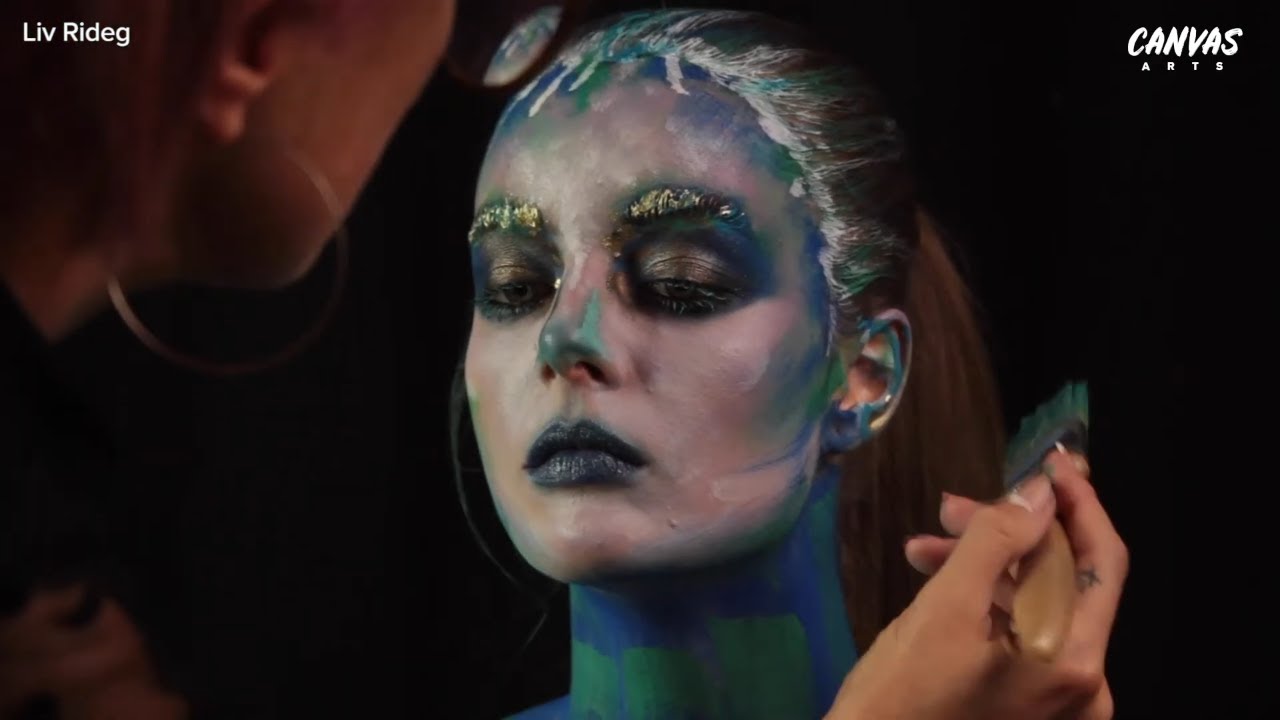In the image, a model is having intricate costume-style makeup applied by an artist, identified as Liv Reidegg, as indicated by the text "Liv Reidegg" in the upper left corner. The brand or platform "Canvas Arts" is visible in the upper right corner. The artist, who has a medium skin tone and wears a large hoop earring in her right ear, uses her right hand to delicately paint the model's face with a brush dipped in green paint. A small tattoo is visible on the artist's index finger. The model's face is a canvas of colors, featuring a white base with highlights in blue and white. Her dramatic makeup includes blue lips, gold-tinged eyebrows, and a hairline painted white. Her hair is sleekly pulled back to reveal more of the artistry. Extending from her face, her neck is painted green with blue accents around the jawline and ear, creating a striking visual contrast. The overall effect is a bold and striking combination of vivid colors seamlessly blended on her skin.